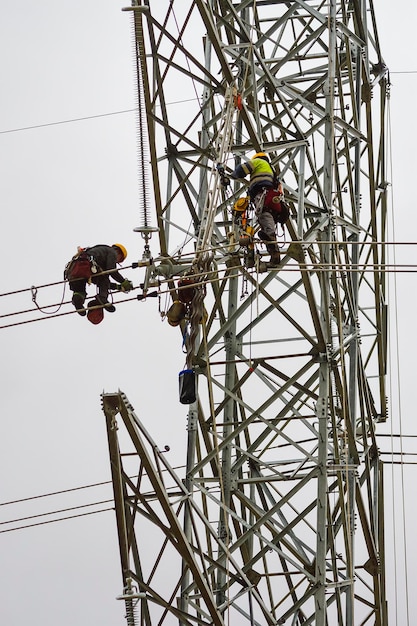In this image, two men are conducting maintenance on a tall, intricate powerline tower that stretches into a gray, almost white sky. The tower, constructed from a complex web of gray tubular metal bars and crisscrossing wires, supports power lines extending out in various directions. One man, positioned on the middle of the tower structure, is standing with a lime green shirt, gray pants, boots, and a tool belt around his waist. His orange hard hat stands out against the metallic backdrop as he works intently. To the left, another worker, dressed in dark clothes and a yellow helmet, is bent over on the top of three horizontal wires, laboring on the wire just below him. He is secured to the line with a rope for safety. Below him, another set of wires extends across the image, with an additional single wire visible at the top. Both men have red packs attached to their hips, which are presumably part of their safety gear, ensuring they remain secure as they meticulously handle the maintenance high above the ground.